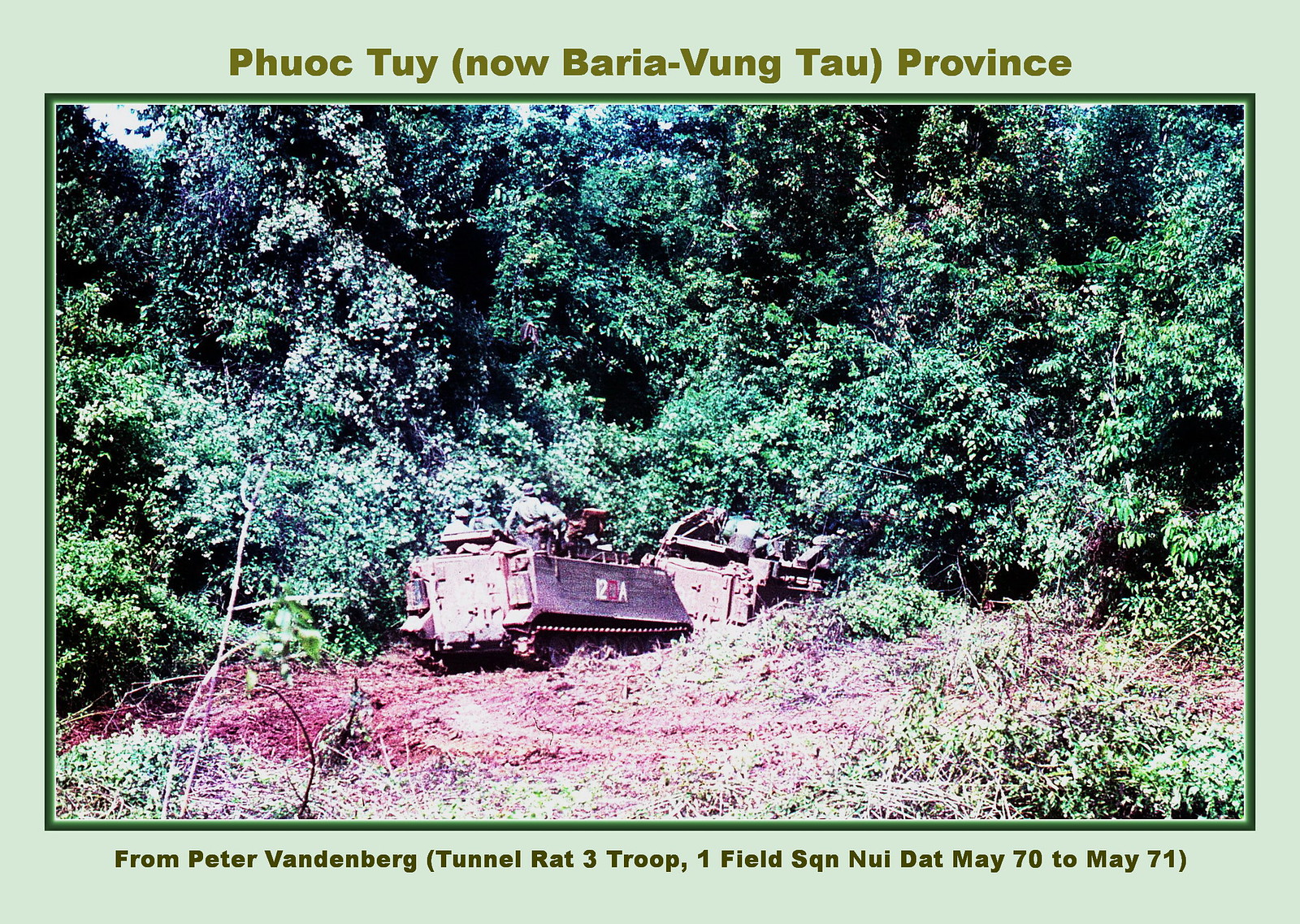This is an older photograph framed with a light green border. At the top in olive green font, it reads "Phu Toi, now Bureau of Vung Tau Province." The bottom of the border is inscribed with, "From Peter Vandenberg, Tunnel Rat, Three Troop, One Field Squadron, Nui Dat, May 1970 to May 1971." The image showcases a dense, forested area with a large canopy of trees. In the foreground, there is a partially cleared space filled with shrubbery and dirt, forming what appears to be a well-trodden path. Positioned on this path are two military vehicles resembling tanks, each equipped with long bases instead of wheels for movement. On closer examination, you can discern soldiers dressed in green uniforms that blend into the surrounding foliage. There are at least four soldiers visible on the rear tank, with likely a similar number on the front vehicle. This detailed depiction captures a moment from a military operation during the Vietnam War era.